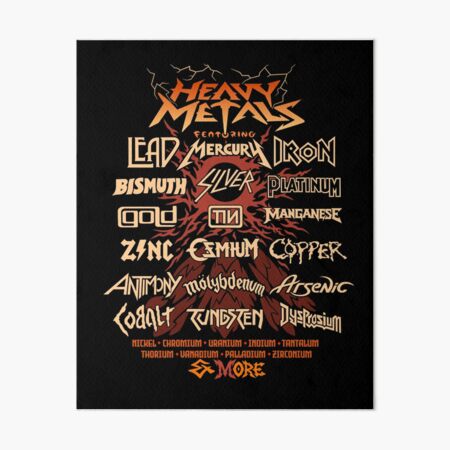The image is an advertisement styled as a concert poster with a black background, prominently titled "Heavy Metals Featuring." It emulates the aesthetic of an 80s rock tour, with the names of various heavy metals presented as if they were band names, each rendered in fonts reminiscent of famous rock and metal bands. Mercury appears in a Metallica-like font, while Tin mimics the Nine Inch Nails logo. Oshzum is written in an Ozzy Osbourne style, and Motley Dunvin channels the Motley Crue look. Tungsten, Iron, and Platinum are styled like Iron Maiden, and Arsenic, Dysprosium, and Manganese take after Def Leppard’s design. Lead, Bismuth, Gold, and Zinc are in a font similar to AC/DC, while Cobalt and Timony are depicted in an off-white color. The background features a striking image of a volcano with an eye peering from the top, adding a dramatic and intense atmosphere to the ad. The metals listed include mercury, lead, iron, bismuth, silver, platinum, gold, tin, manganese, zinc, copper, molybdenum, arsenic, cobalt, tungsten, and dysprosium, all detailed as if they were part of a grand, metallic concert lineup.